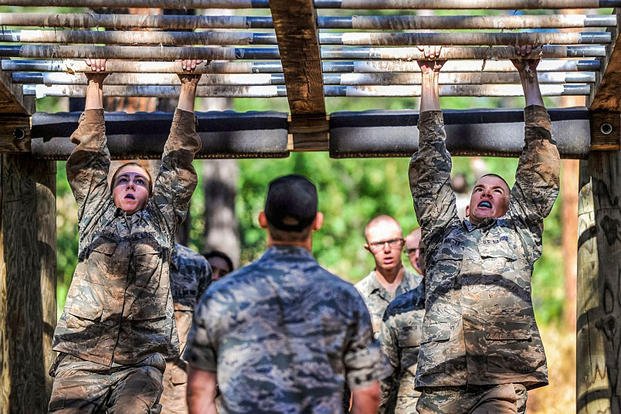In this photograph, likely taken during an Air Force boot camp, we see recruits engaged in a rigorous obstacle course set outdoors, surrounded by green-leafed trees. Centered in the image are two soldiers—a man on the right and a woman on the left—both dressed in camouflaged fatigues and appearing muddy, suggesting they recently navigated a challenging terrain. They hang from overhead monkey bars, gripping them firmly with both hands while concentrating intently on their task. The man on the right looks particularly distressed. In the foreground stands an instructor, back to the camera, wearing a black hat and a gray camouflage shirt. Behind the hanging recruits, there is another instructor with glasses observing the scene, mouth open and appearing apprehensive. Additional soldiers, at least three, wait in line to tackle the monkey bars, their figures blurred against the backdrop of lush foliage. The sky suggests mid-evening conditions, casting shadows across the obstacle course.